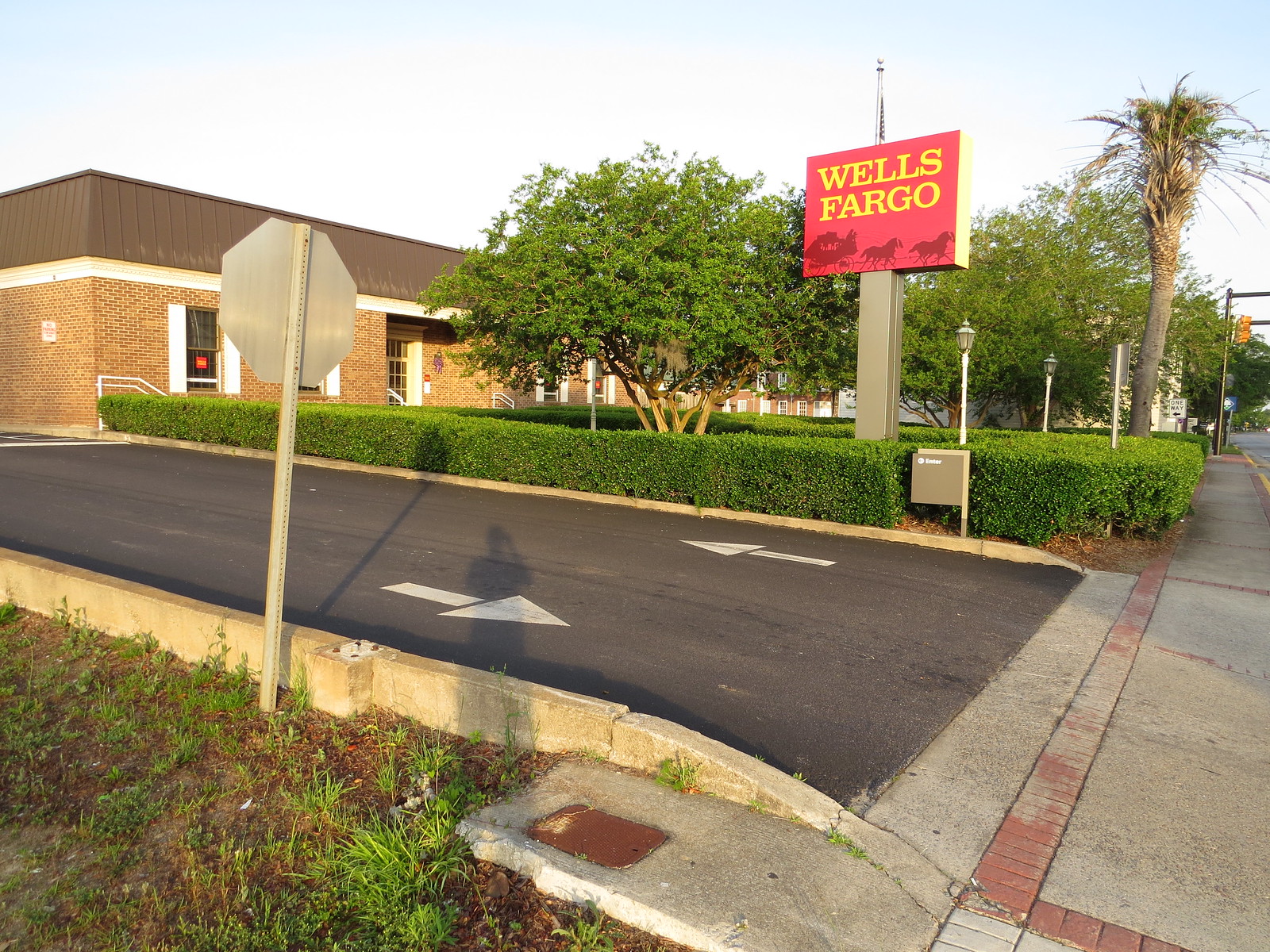The photograph captures the entrance to a Wells Fargo bank on a bright sunny day. Dominating the scene is the Wells Fargo sign, featuring a red background and yellow font, along with a dark red silhouette of a cart pulled by two horses. This sign is mounted on a large brown metal pole situated behind some hedges. The entrance comprises an asphalt two-way driveway with white directional arrows painted on it, bordered by curbs. Adjacent to the driveway is a gray sidewalk lined with slightly faded red brick. The surrounding area includes grass patches, a stop sign amidst some sprouting grass shoots, and a brown brick building housing the bank. Traffic lights and light posts with multiple bulbs are visible along the street. The landscape is further adorned with palm trees and other trees in the distance. The sky above is a clear blue, reflecting the bright, sunny daytime setting.